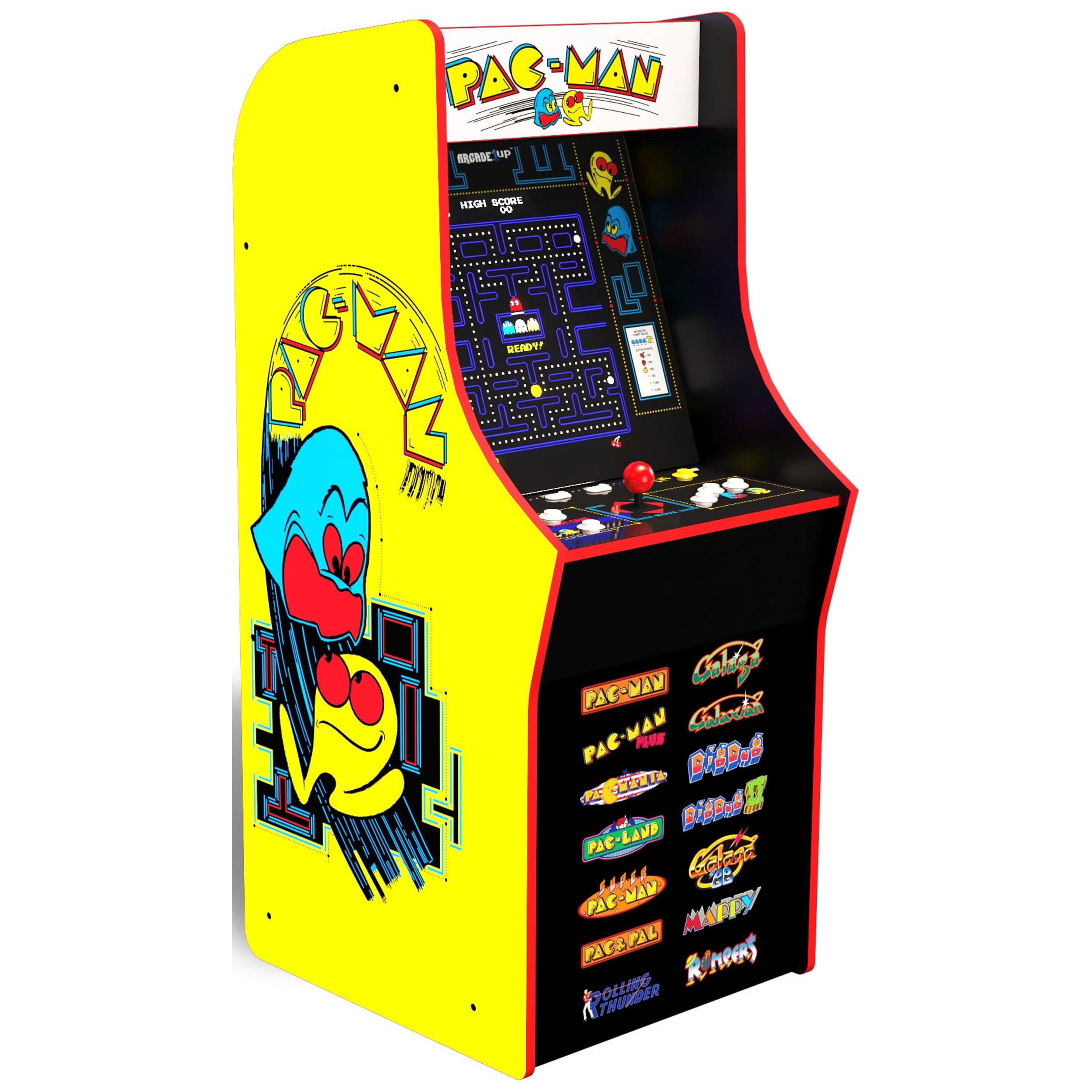This image features a classic Pac-Man arcade machine captured from a slightly leftward angle, showcasing both the side and front panels. The machine's design prominently includes vibrant hues of yellow, red, light blue, dark blue, green, black, and neon blue. The left side panel of the arcade cabinet is a solid yellow, with "Pac-Man" written in an arched style about one-third down the panel. Below this, a blue ghost with red eyes and mouth faces a yellow character, also with red eyes and legs, set against a high-tech looking black, red, and blue backdrop.

At the top of the front panel, "Pac-Man" is displayed in various styles and designs. The control panel features a red joystick and white buttons. The game screen, which appears to be powered on, displays the iconic blue maze with Pac-Man, represented by a yellow circle with a mouth, navigating the maze while avoiding or chasing colorful ghosts, depending on whether he has consumed one of the maze's power pellets. Below the screen, there are additional game names listed in two columns of six rows, indicating multiple playable games on the machine.